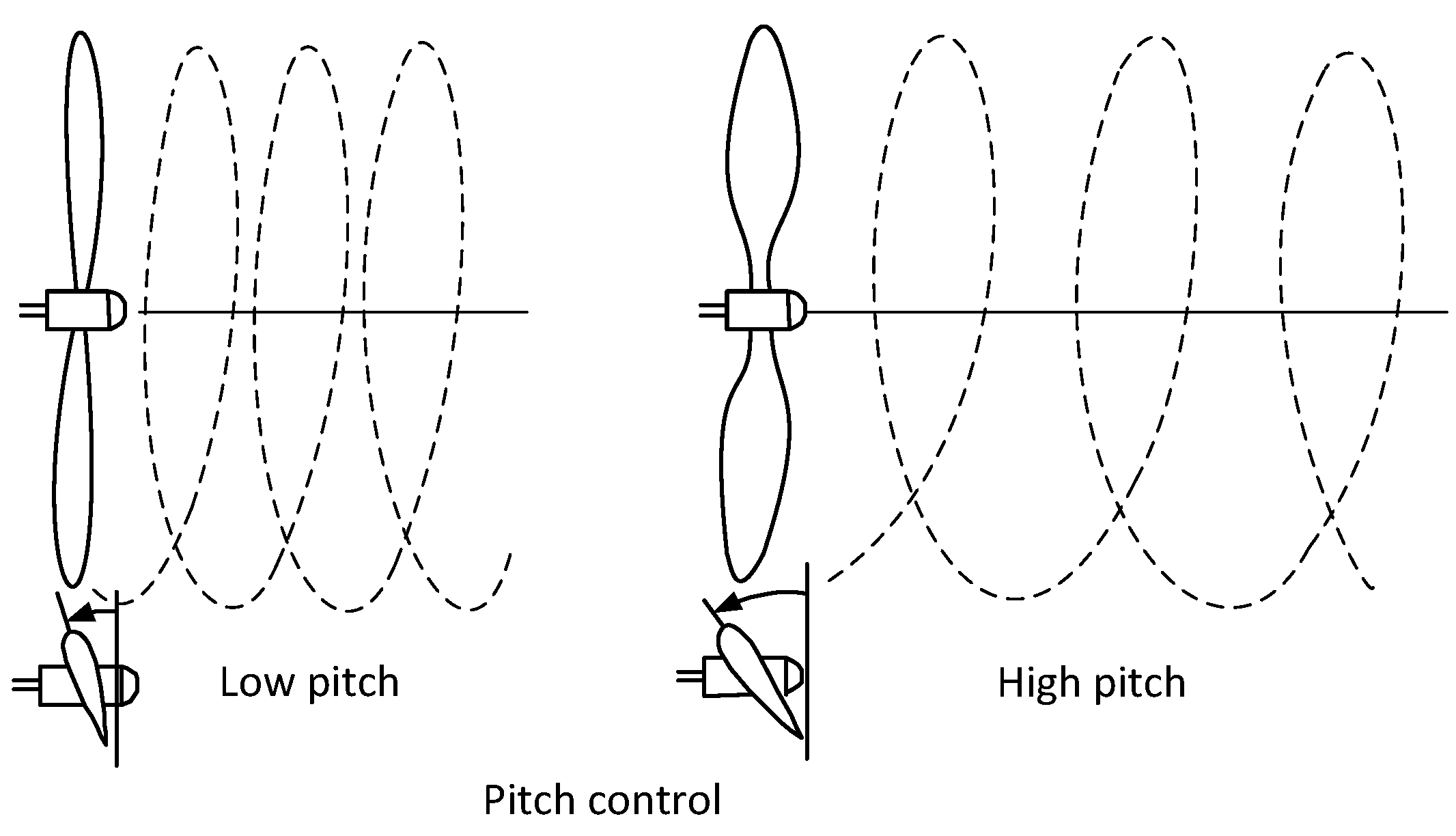This image is a detailed black-and-white diagram titled "Pitch Control," commonly seen in scientific papers or textbooks. The diagram features two distinct sections, each illustrating different pitch settings of a fan-like propeller.

On the left side, a propeller with smaller blades is depicted, around which narrow spirals are generated, symbolizing low pitch. Below this, "Low Pitch" is labeled, and a control dial is positioned towards the center-right, indicating the setting for low pitch.

To the right, a similar diagram shows a propeller with larger blades generating wider spirals. This section is labeled "High Pitch," with its dial positioned further down, towards the center-left, signifying the high pitch setting.

The bottom middle of the image prominently displays the term "Pitch Control," encapsulating the function of the depicted mechanisms. The diagram effectively contrasts the low and high pitch settings through the differences in blade size and spiral spacing, accompanied by control dials that adjust the pitch accordingly.